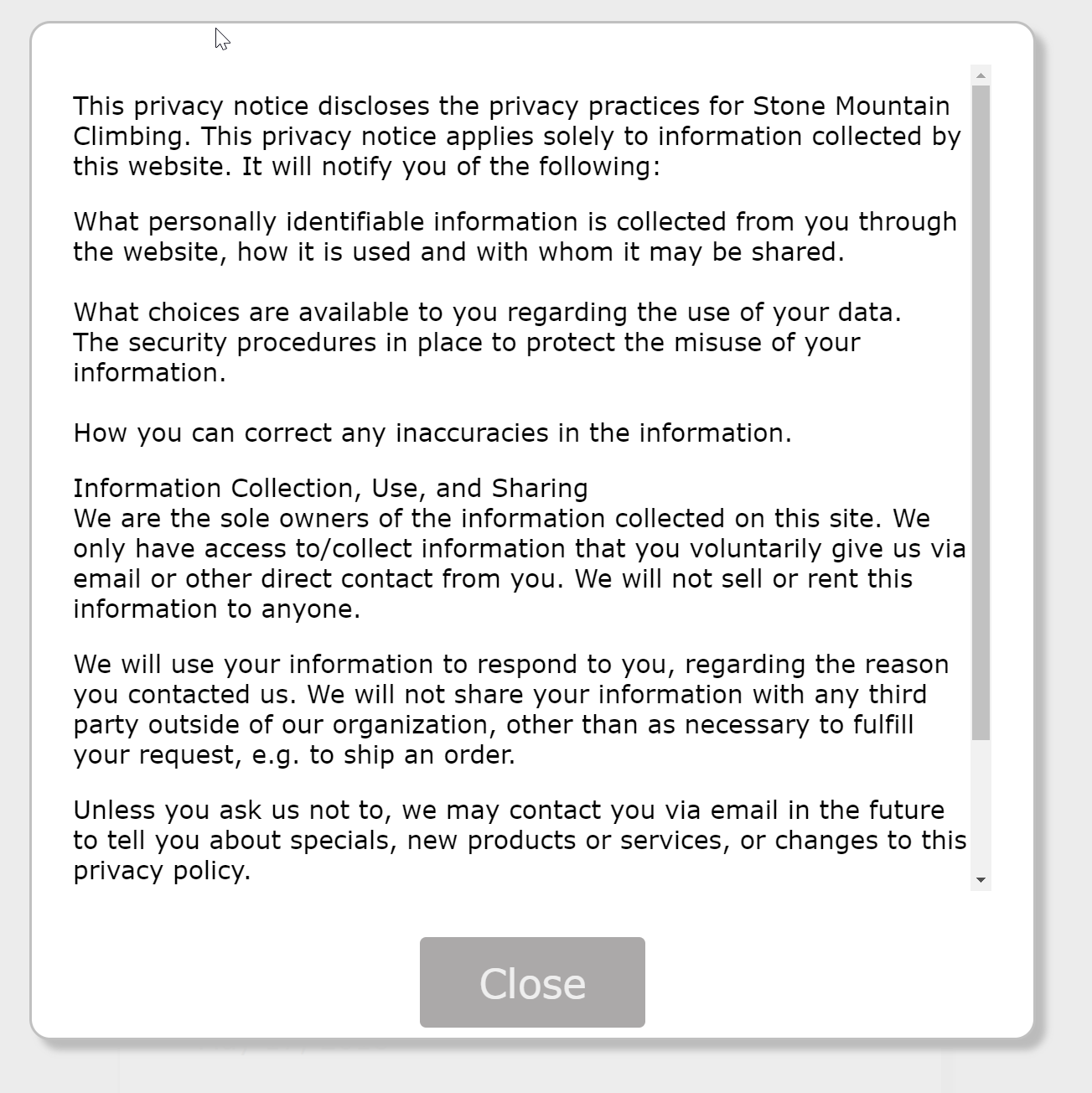The image depicts a screenshot of a webpage, captured from either a laptop or desktop computer. The screenshot features two distinct sections: a light baby blue background and a central white box with rounded corners. 

In the upper section of the white box, a small white mouse pointer is visible. Below this pointer, there is a paragraph in black font, separated by lines. The paragraph is a privacy notice that reads:

"This privacy notice discloses the privacy practices for Stone Mountain Climbing. This